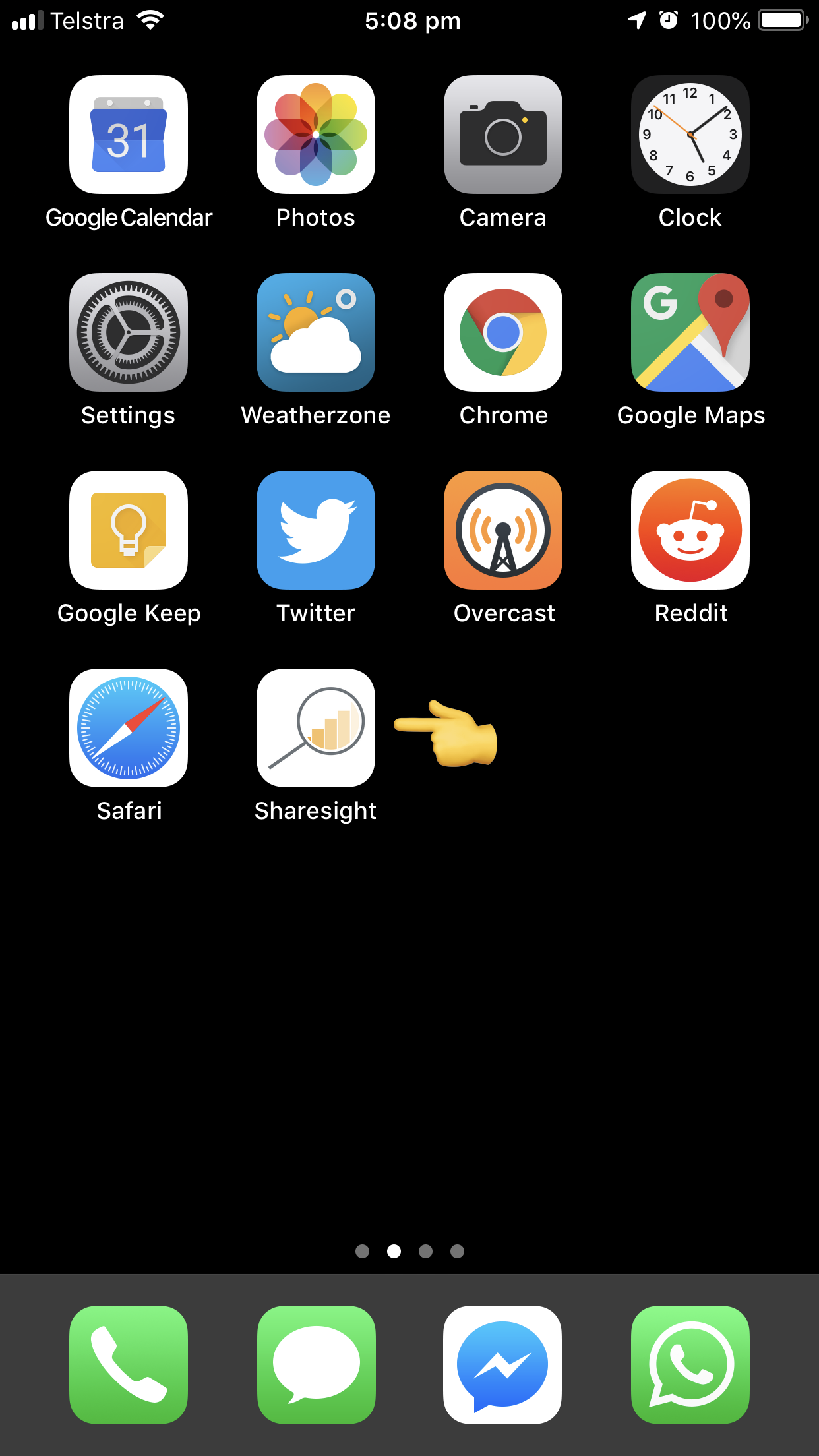This is a detailed screenshot of an iPhone's main screen, captured in dark mode. The status bar at the top displays the cell service provider, Telestra, with full Wi-Fi signal, and it shows the phone is fully charged at 100%. It’s 5:08 p.m., and an alarm is set, indicated by the clock icon.

Prominently featured in the screenshot is a finger-pointing emoji highlighting the 'Share Site' app, suggesting the user is guiding someone on its location. Other visible apps on this screen include Google Calendar, Photos, Camera, Clock, Settings, Weather Zone, Google Chrome, Google Maps, Google Keep, Twitter, Overcast, Reddit, Safari, and the highlighted Share Site.

The screenshot also reveals that this is the second of four home screen pages, hinted by the page indicator at the bottom. The dock at the bottom holds the Phone app, Messages shortcut, and WhatsApp, providing quick access to these frequently used applications.